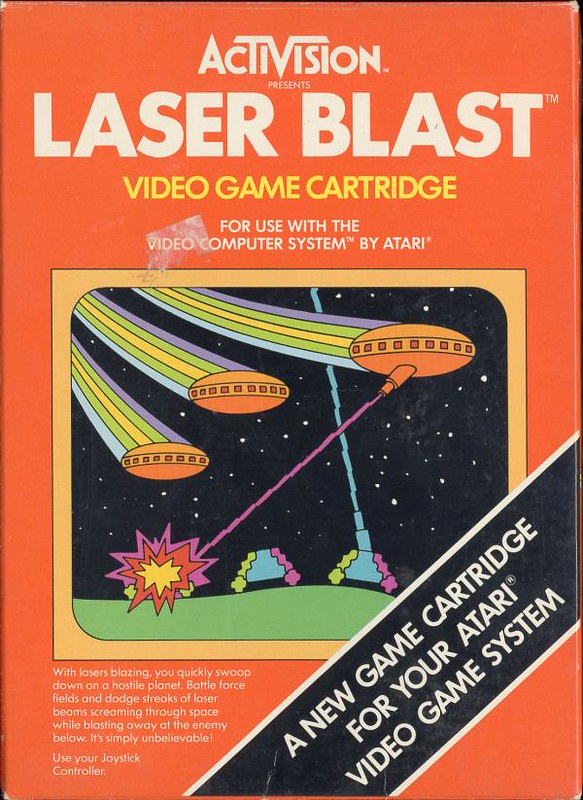The image is a photograph of vintage video game packaging for "Laser Blast," produced by Activision for use with the video computer system by Atari. The box has a striking orange background. At the top, the text "Activision presents Laser Blast" is displayed prominently in white, while below that, "video game cartridge" is written in yellow, and "for use with the video computer system by Atari" appears in white. 

Centrally, there's a framed illustration trimmed in light orange depicting a night sky where three UFOs, appearing in orange, swoop down towards the ground. The UFOs are engaged in a fierce battle, sending streaks of laser beams zapping towards two tanks below, one of which is already obliterated and in flames. Diagonally across the center of the box is a black banner with white text that reads, "A new game cartridge for your Atari video game system." The depiction of the action scene with laser beams and spaceships epitomizes the intense sci-fi gameplay experience that the cartridge promises.